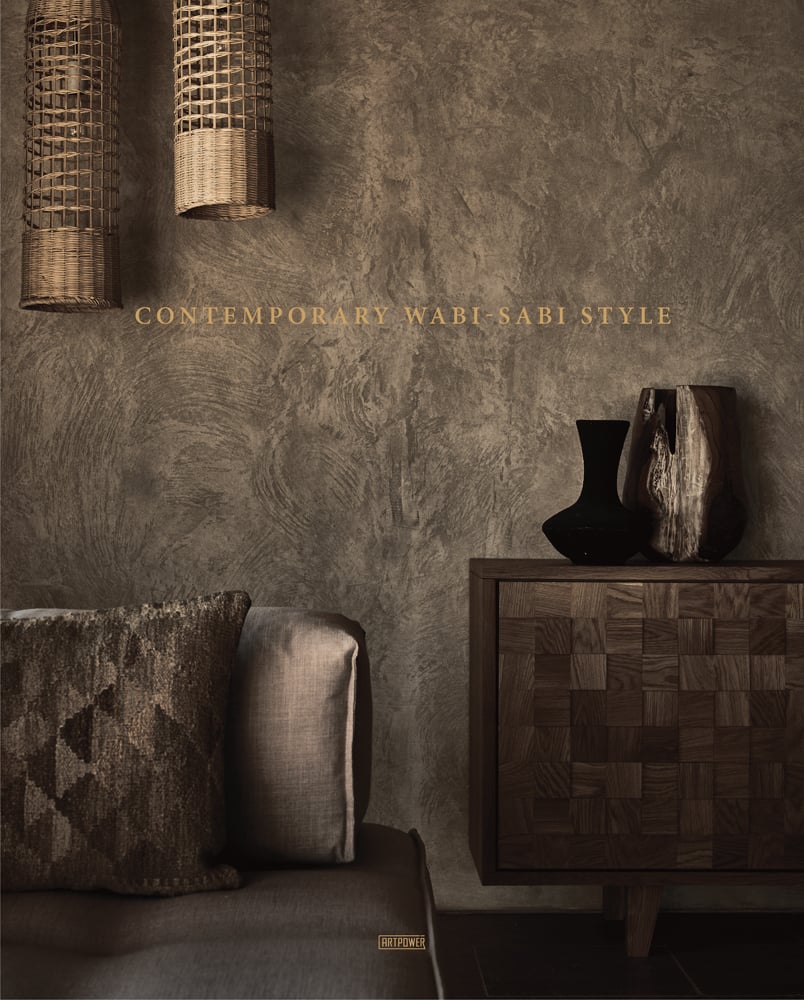This photograph depicts the interior of a room characterized by a contemporary Wabi-Sabi aesthetic, highlighted by text in the center of the image that reads "CONTEMPORARY WABI-SABI STYLE" in bold yellow letters. Below, also in yellow, are the words "Art Power." The room features a grey wall adorned with two cylindrical decorative items made of woven wooden sticks, adding a natural, rustic touch. In the bottom left corner, a partial view of a grey couch is visible with a light brown pillow featuring a triangular design. To the right, a small black table on the floor supports a black pot and another decorative sculpture. The space is meticulously arranged, showcasing a blend of minimalist and natural elements typical of the Wabi-Sabi style.